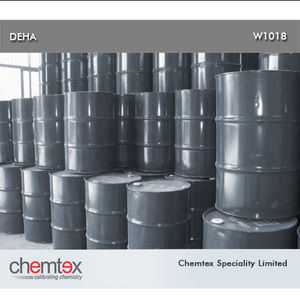The image depicts a monochromatic industrial setting with a stack of dark gray, metallic barrels arranged in three distinct tiers. The bottom tier juts out the furthest, followed by the second row, and the top tier slightly recessed. The warehouse background, including the floor and a window frame off to the left, all contribute to the grayscale appearance of the scene. A light gray banner spans across the top of the image, featuring "DEHA" on the left and "W1018" on the right, both rendered in white text. At the bottom, the company’s logo is displayed: on the left, "Chemtex" written in black font with red 'E's and the tagline "Calibrating Chemistry" beneath it; on the right, "Chemtex Specialty Limited" on a light gray background. The composition suggests a corporate or safety-related presentation slide for the company Chemtex.